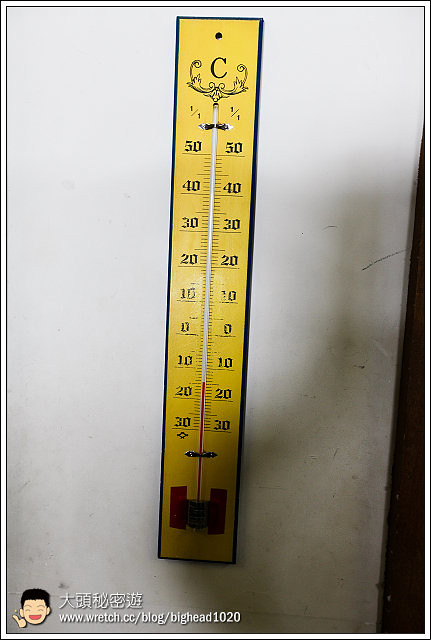The photograph captures a vintage thermostat prominently mounted on a white wall. The thermostat features a wooden base, painted a bright yellow, with intricate black ink detailing. At the top, the letter "C" signifies that the device is calibrated in Celsius. Surrounding the "C," a delicate filigree flourish adds an ornate touch, extending from its left side, curling beneath, and continuing to the right side.

The central glass tube of the thermometer is encased and secured by three metal fasteners: two small ones at the upper part and a larger one at the bottom. Flanking the top corners of the glass tube are the markings "1/1" on each side. The numerical temperature scale runs vertically down both sides of the thermometer, marked at intervals: 50, 40, 30, 20, 10, 0, -10, -20, -30. The mercury inside the thermometer, indicating the current temperature, sits at -15 degrees Celsius.